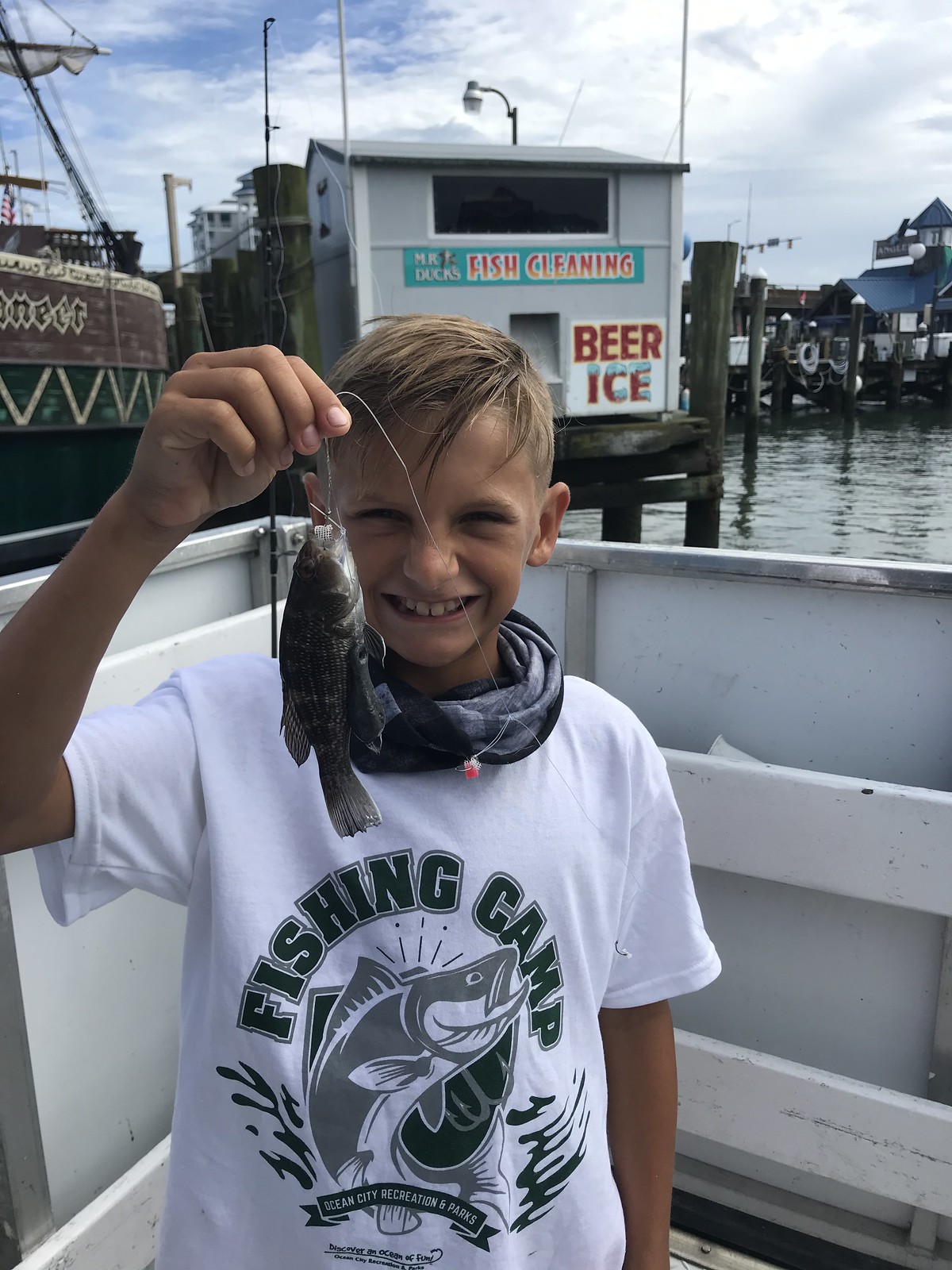In this wholesome image, front and center is a young boy with blonde, slightly wet hair, combed to the right side, wearing a white T-shirt that says "Fishing Camp" with a jumping fish depicted on it. He sports a scarf bandana around his neck and beams proudly as he holds a tiny, dark-colored smallmouth bass with a hook still in its mouth in his right hand. The boy is standing on what appears to be a boat, indicated by the boat's wall coming up just behind his head. The scene is set on an overcast day with clouds in the sky, adding to the tranquil atmosphere. Behind him, there is a tall brown boat and a white square building on the pier with a banner that reads "Beer Ice Fish Cleaning." To the right side of the image, the lake water and portions of other boats and piers are also visible.